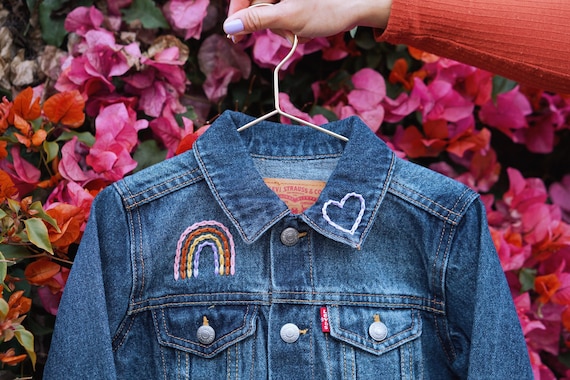In the image, a woman's arm, adorned in an orange sweater, extends from the top right of the frame, holding the white metal hook of a hanger. This hanger supports a child's blue denim jacket, which is detailed with an embroidered rainbow on the right side of the chest and a white heart on the left side of the collar. The woman's thumb is painted with blue nail polish. The background is a vibrant array of pink, red, and coral flowers. The usual metal buttons typical of a denim jacket are visible, adding to the detailed description of the garment.